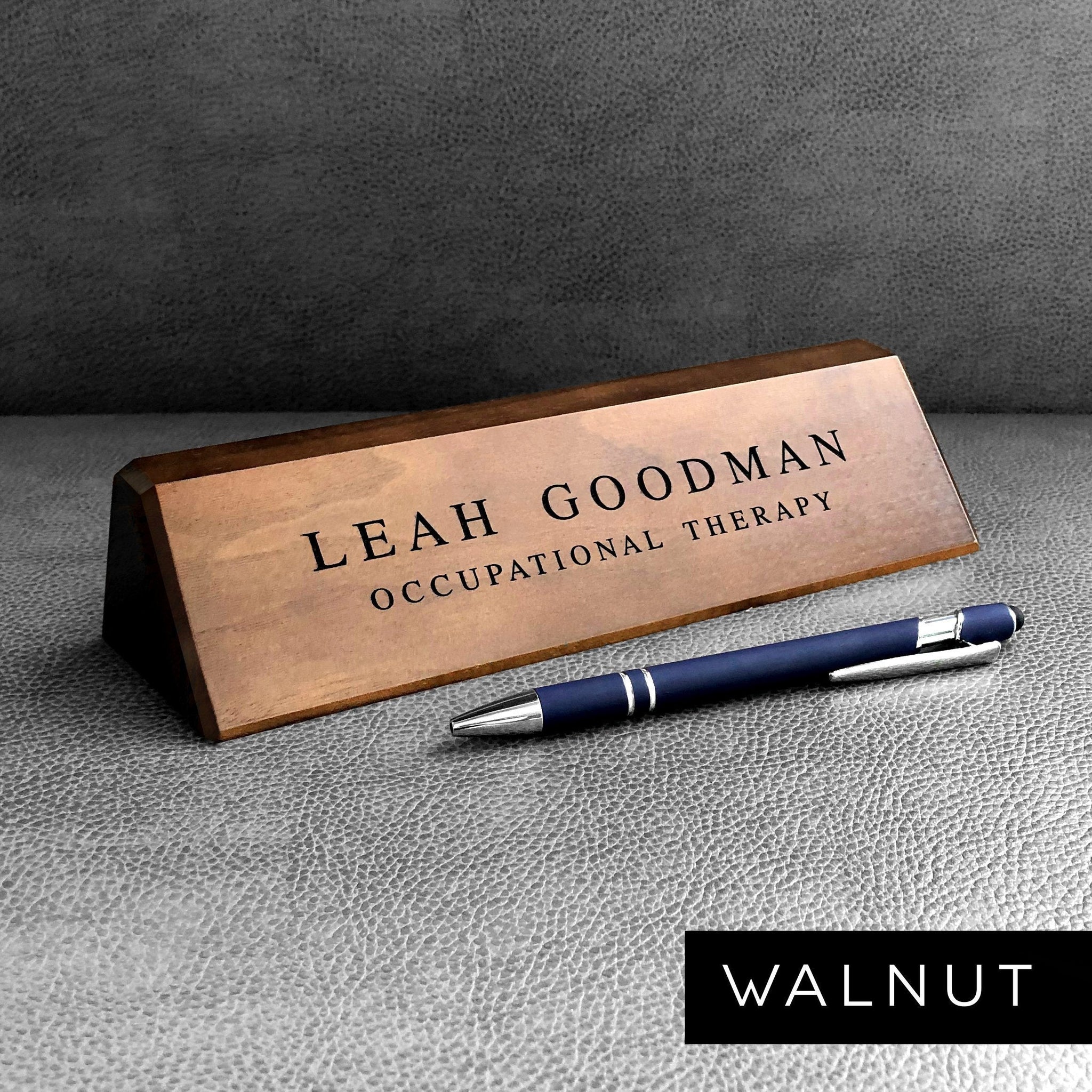The photograph showcases a wooden name plaque with a carved inscription reading "Leah Goodman, Occupational Therapy." The plaque, stained in a dark brown hue, possibly walnut, features the grain of the wood prominently. The name is engraved in black, while "Occupational Therapy" appears beneath it. Adjacent to the plaque lies a blue pen with a silver tip and clip. The scene is set against what appears to be a gray leather car seat, with minimal color contrast. In the lower right corner of the image, a black rectangle contains the word "Walnut," suggesting the type of wood used for the plaque.